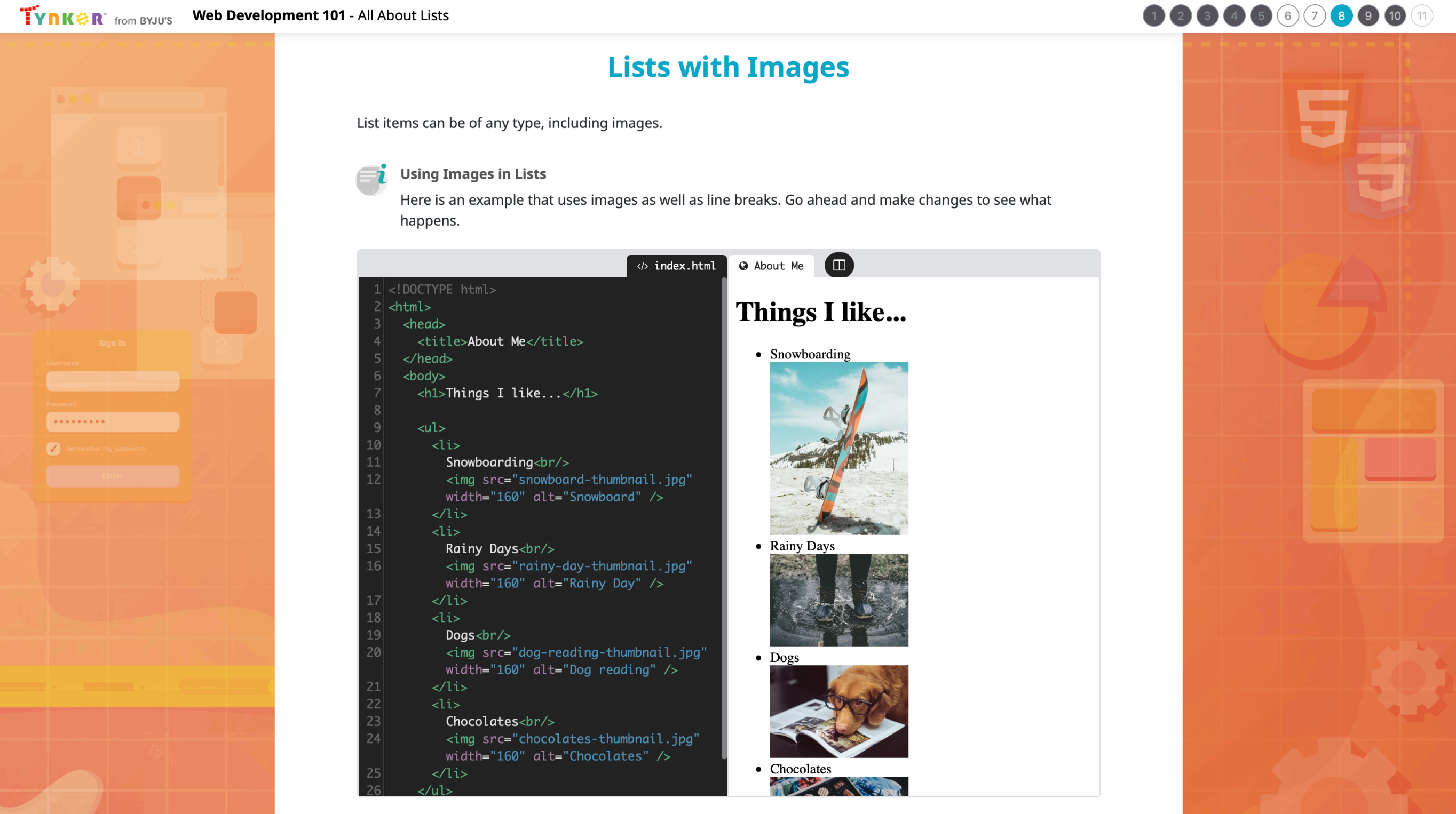This image represents various aspects of web development, focusing on the project 'TriCore'. It showcases the use of lists and images under different modules such as 'AllAboutList' and 'ListsWithImages'. The caption provides visual representation with an example demonstrating images and line breaks. 

In the central portion of the image, there is a section titled "Things I Like" with items listed such as 'RainyDays', 'Drugs', and 'ChessSolid'. The color scheme features an orange gradient, with lighter orange segments on both the left and right sides, and a darker orange on the right side. 

The middle section has a clear white background, divided into two distinct parts. On the left, there is a black square displaying code snippets typical in web development. On the right, a white square showcases web page images, illustrating how images can be embedded within lists for enhanced visual presentation.